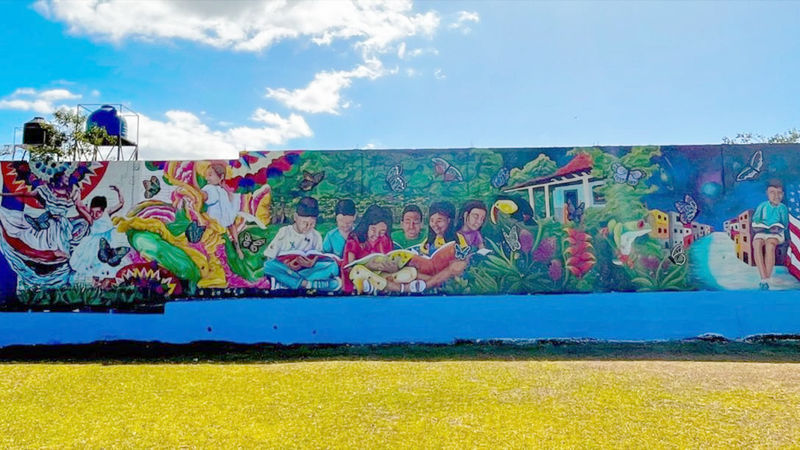This vibrant mural spans the side of a long white concrete wall set against a backdrop of a clear blue sky with fluffy white clouds. In the foreground, a lush green grass field stretches out. The mural starts on the right side with a young person sitting on a building, engrossed in a book beside an American flag. Butterflies flit about in this section, which also features bright red and purple flowers and a striking black and yellow bird. Adjacent to this, a scene unfolds with children sitting on the ground, reading books amidst trees and more butterflies, suggesting a peaceful, nature-filled setting. Transitioning further left, the mural depicts lively dancers — a Mexican woman in a colorful, fluffy skirt twirling around and another dancer in a red and white dress. The entire artwork is infused with elements of nature, community, and vibrant colors, creating an engaging piece of street art that beautifully adorns the urban landscape. In the distant background on the left, two towers with water containers are visible, adding to the rich context of this downtown city area.